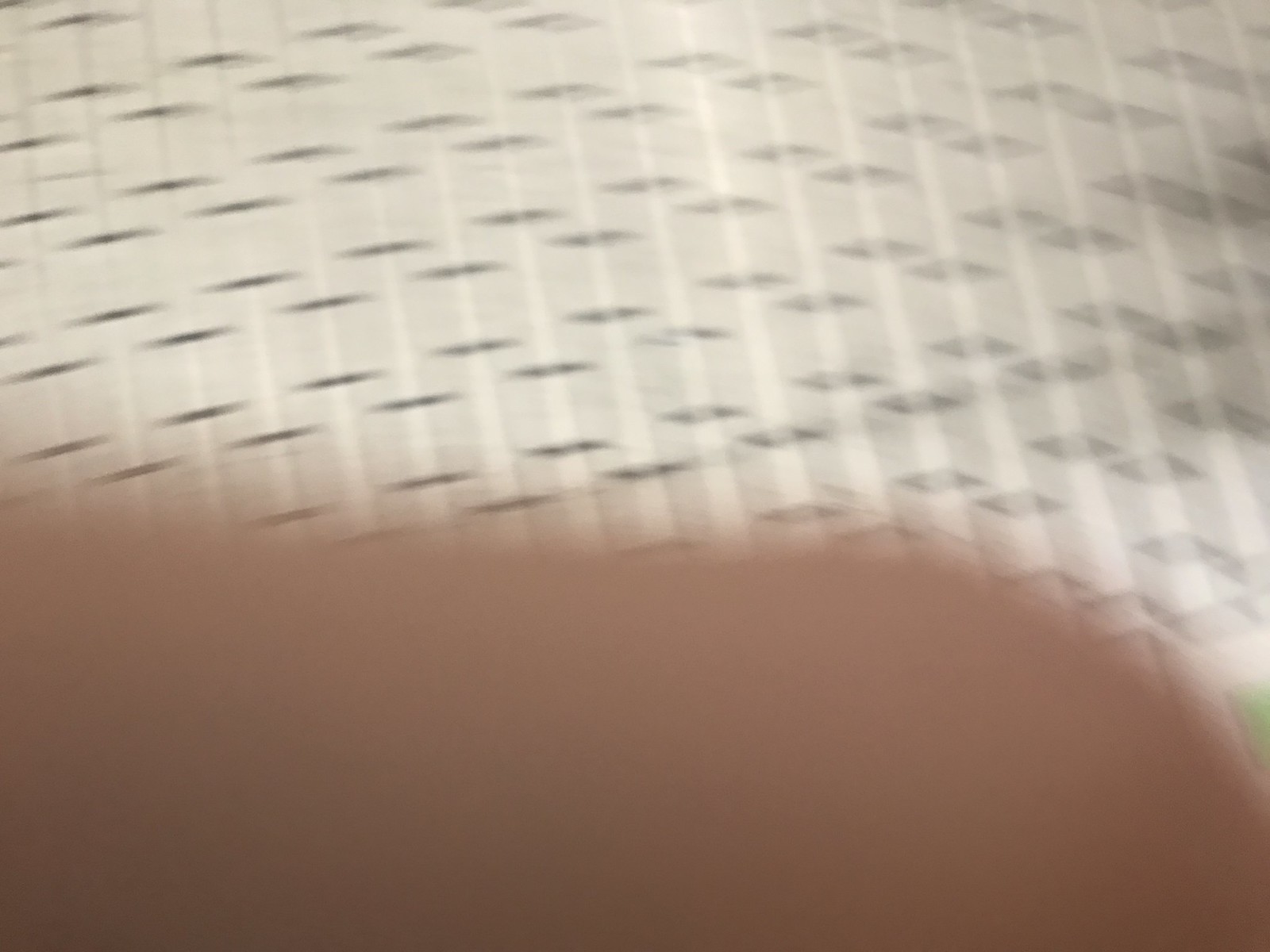This image captures a close-up of a textured material that appears to be either fabric or paper. The surface is predominantly white, adorned with delicate black lines running across it. The material has been carefully folded in an accordion-like fashion, creating small, evenly spaced ridges that resemble the pleats of a paper fan. As the eye moves towards the right side of the photo, the straight black lines transform into a pattern of small diamonds. This intricate design adds an element of visual interest and complexity to the image. The bottom part of the photo is partially obscured by the photographer's finger, which inadvertently blocks the lens, adding an unintended yet human touch to the composition.